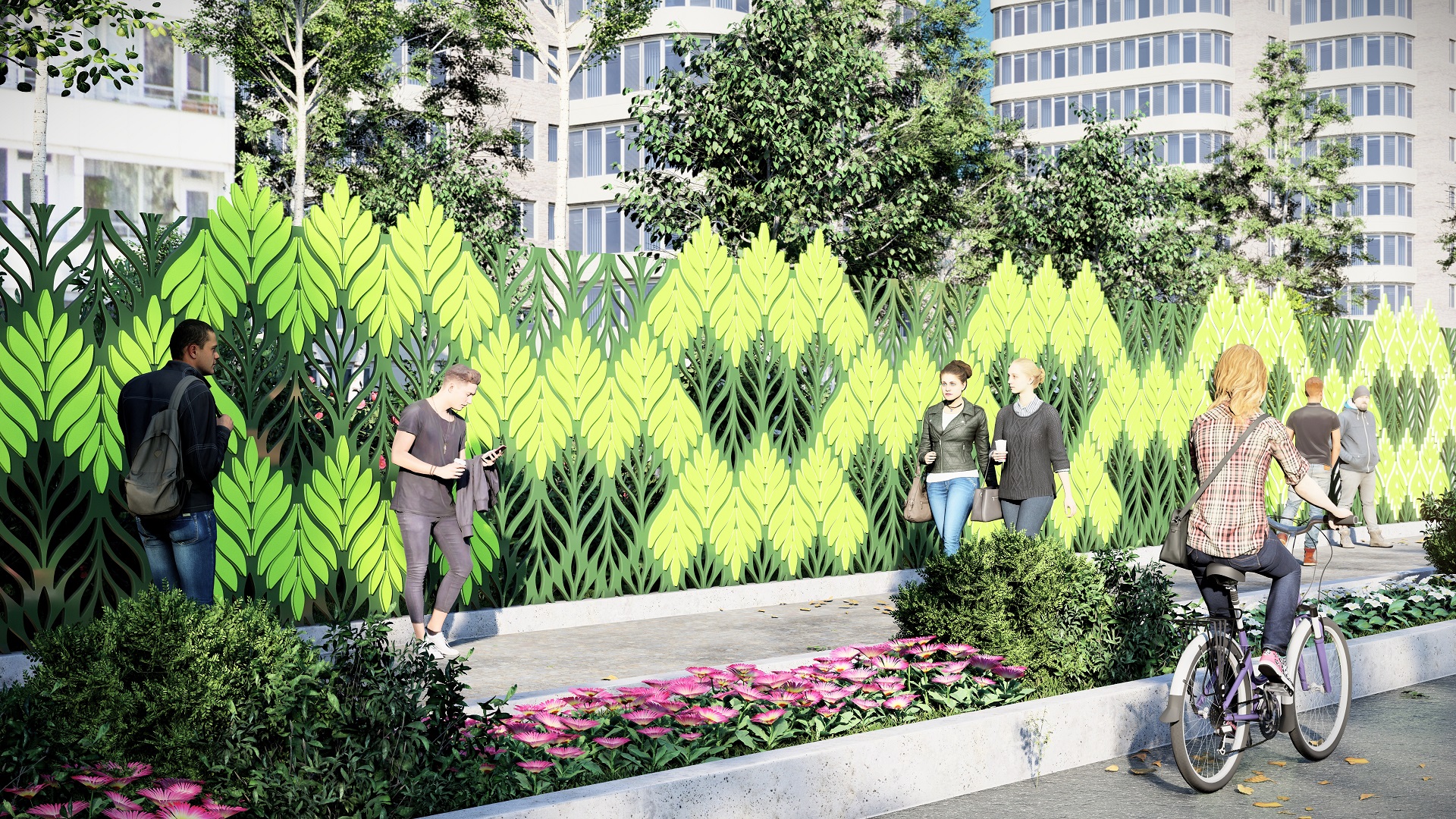In this vibrant scene, an uncanny, stylized group of 3D-like human figures populates the area, evoking an eerie realism. The sidewalk, stretching across the foreground, features several people walking and standing. Prominently visible on the bottom left side is a black man with a gray backpack. Nearby, a man leans against an intricate, dark green fence with lighter green flower patterns arranged in a zigzag across it, engaged with his cell phone. Walking towards the left, two women appear, one clad in a black leather jacket and light blue jeans, and her companion in a black shirt with blue jeans.

Dominating the right side of the image is a woman riding a pink bicycle with white fenders down the street. She sports a red-and-white plaid shirt with sleeves rolled up just above her elbows and blue jeans. Her blonde hair cascades just below her shoulders, and a purse hangs over her shoulder down to her hip.

The sidewalk features a concrete barrier lined with vibrant pink flowers and lush green foliage. Beyond the intricate fence, tall, verdant trees rise, giving way to a backdrop of towering white buildings adorned with blue windows. The unique blend of artificial and natural elements, combined with the stylized figures, creates a strikingly detailed and immersive scene.